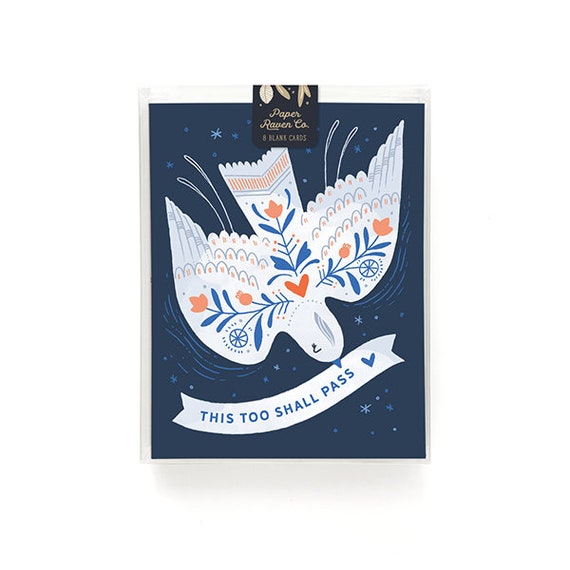The image depicts a vertical condolence card featuring a beautifully illustrated white dove in mid-flight, descending with its wings spread wide. The dove is adorned with intricate orange flowers, blue leaves, and orange hearts, intricately painted into the feathers of its wings and tail. In the dove's blue beak, it carries a delicate white ribbon inscribed with the comforting message, "This too shall pass," in deep blue lettering. The background of the card is a rich navy blue, dotted with an array of lighter blue stars, adding a serene and hopeful atmosphere to the design. The card is part of a set labeled "eight blank cards," providing ample space for personal messages of empathy and support.